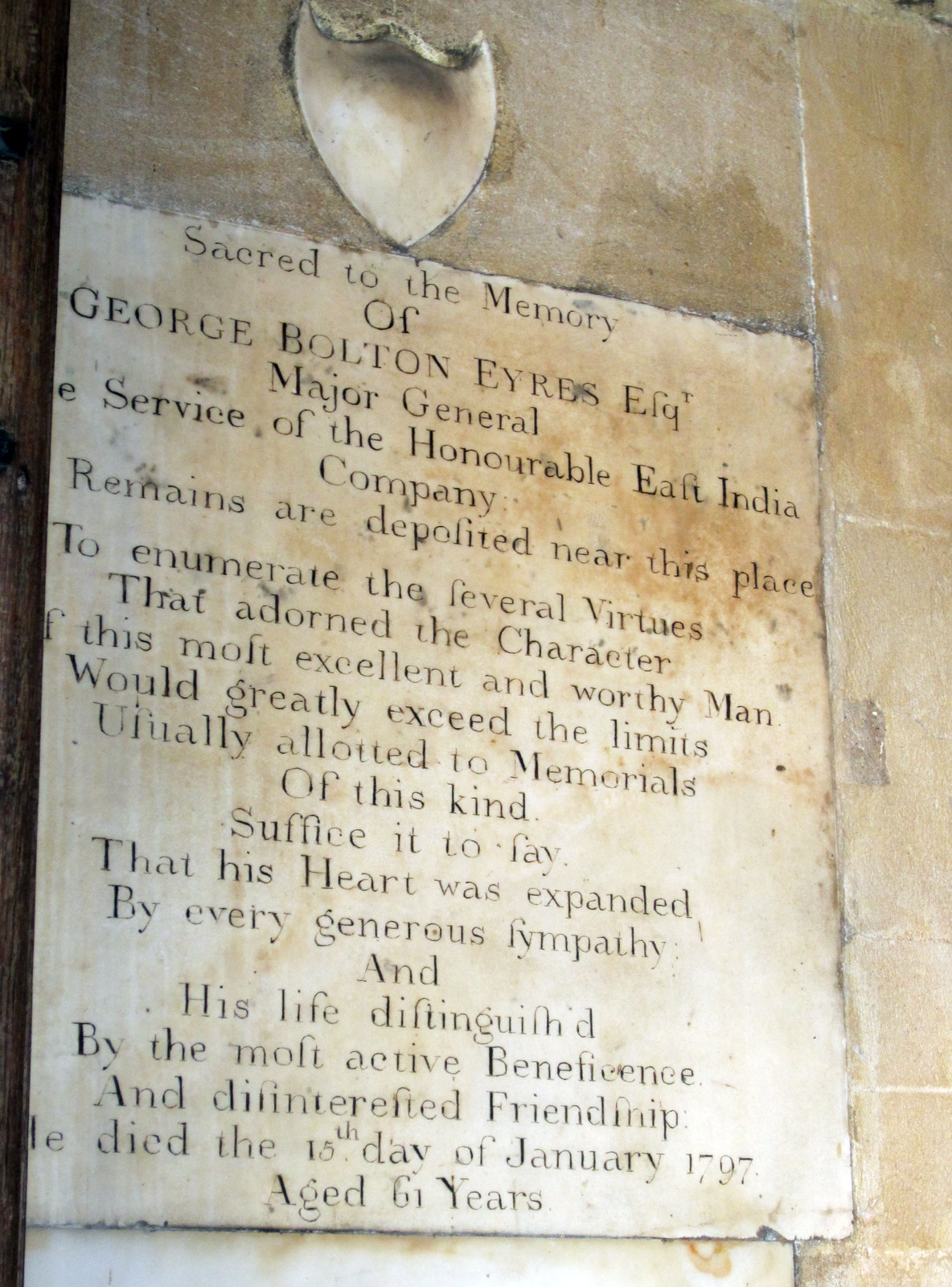The image captures an old, weathered concrete or stone wall, likely part of a building, which could either be inside or outside. The wall comprises large, plain sections, white or light brown in color. Set into this wall is a stone plaque dedicated to the memory of George Bolton Ayers, Esquire, a Major General in the service of the Honorable East India Company. The plaque is distinguished by an embossed shield at the top, which frames the text below. The inscription details that the remains are deposited near this spot and attempts to convey the virtues of this esteemed and worthy man. It reads: "Sacred to the memory of George Bolton Ayers, Esquire, Major General, Service of the Honorable East India Company. Remains are deposited near this place. To enumerate the several virtues that adorned the character of this most excellent and worthy man would greatly exceed the limits usually allowed to memorials of this kind. Suffice it to say that his heart was expanded by every generous sympathy and his life distinguished by the most active beneficence and disinterested friendship. He died the 15th day of January 1797 at the age of 61 years." The text features the use of the long "s," resembling an "f" without the cross stroke. This photograph is taken from a slightly low and leftward angle, giving just a hint of the age and gravitas of the commemorative stone.